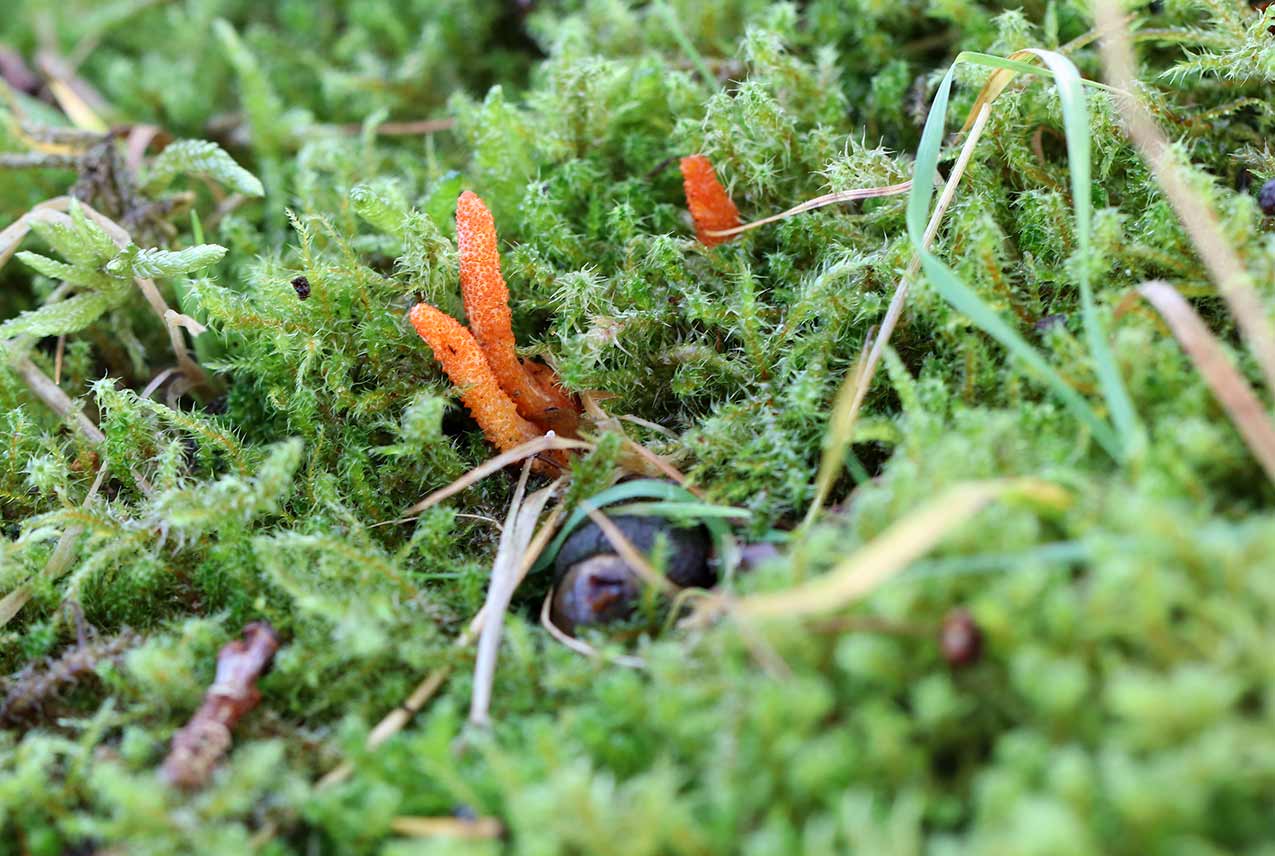This detailed photograph captures a close-up view of a vibrant natural scene, likely taken during daylight outdoors, featuring a diverse array of tiny plants and vegetation. The image heavily focuses on a dense cluster of green, spiky moss-like plants with a soft, fuzzy texture. Amidst the greenery, three prominent orange, plant-like structures stand out in the picture's center, likely botanical growths or perhaps even cordyceps. Scattered among the moss are a few brown and green grass blades, some of which are wilted and folded over.

Adding to the complexity of the scene, there are several small twigs, branches, and possibly a dark brown rock or piece of wood nestled among the plants. The image has a selective focus, with the center being the sharpest point, showcasing the orange structures, while the foreground and background are slightly blurred. This selective focus creates an intriguing depth, with muted yet vibrant tones of green, orange, brown, and hints of a purple-y brown color. The combination of these elements suggests a rich, micro-ecosystem thriving either in a natural setting or a cultivated garden space. No animals or human elements are present, and there is no text on the photograph, immersing the viewer entirely in the lush, intricate plant life.